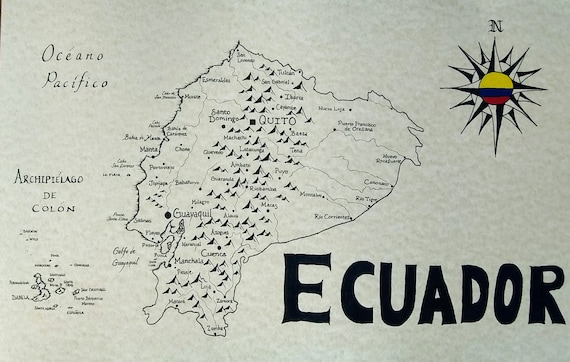This is an in-color landscape photograph of a detailed, sketch-style map of Ecuador. The map prominently features big, bold, black letters reading "Ecuador" in a cubist typeface in the bottom right corner. A compass marked solely with an "N" for north, styled with the colors of the Ecuadorian flag—yellow, blue, and red—adorns the top right corner, featuring a distinctive pufferfish-like shape beneath it. On the upper left side, the map labels the Pacific Ocean ("Oceano Pacifico"), and below that, it identifies the Galápagos Islands as "Archipelago de Colón." The central portion of the map showcases a drawn representation of the Andes Mountain range running from north to south. The Andes, along with various cities—most notably Quito and Guayaquil—are displayed, though the landmass holds too many place names to list. On the lower left side, some smaller islands, part of the Archipelago de Colón, are depicted but their names are too small to read. The background of the map features a grayish, off-white color, adding to its sketched and slightly textured appearance.